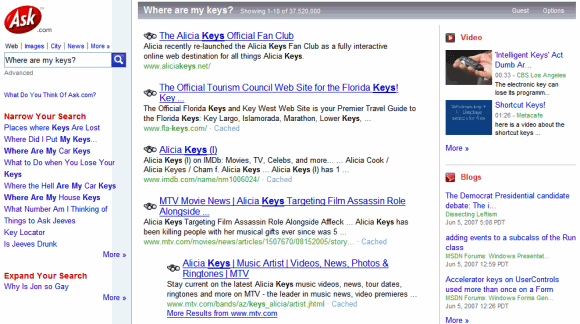The image displays a web page from Ask.com, showcasing various search results related to Alicia Keys and the Florida Keys. Prominently featured is the Alicia Keys official fan club, which has been recently relaunched as a fully interactive online web destination dedicated to all things Alicia Keys. Additionally, the search results include the official tourism website for the Florida Keys and Key West, highlighting it as a premier travel guide. Another result mentions Alicia Keys’ involvement in the film industry, specifically her upcoming role in an assassination film alongside Ben Affleck. A brief historical note is included, stating that Alicia Keys has been captivating audiences with her musical talents since the age of 5. Alongside these results, there are blog entries about the Democratic presidential candidates' debate dates from June 5, 2007, and technical terms related to user controls and accelerator keys.